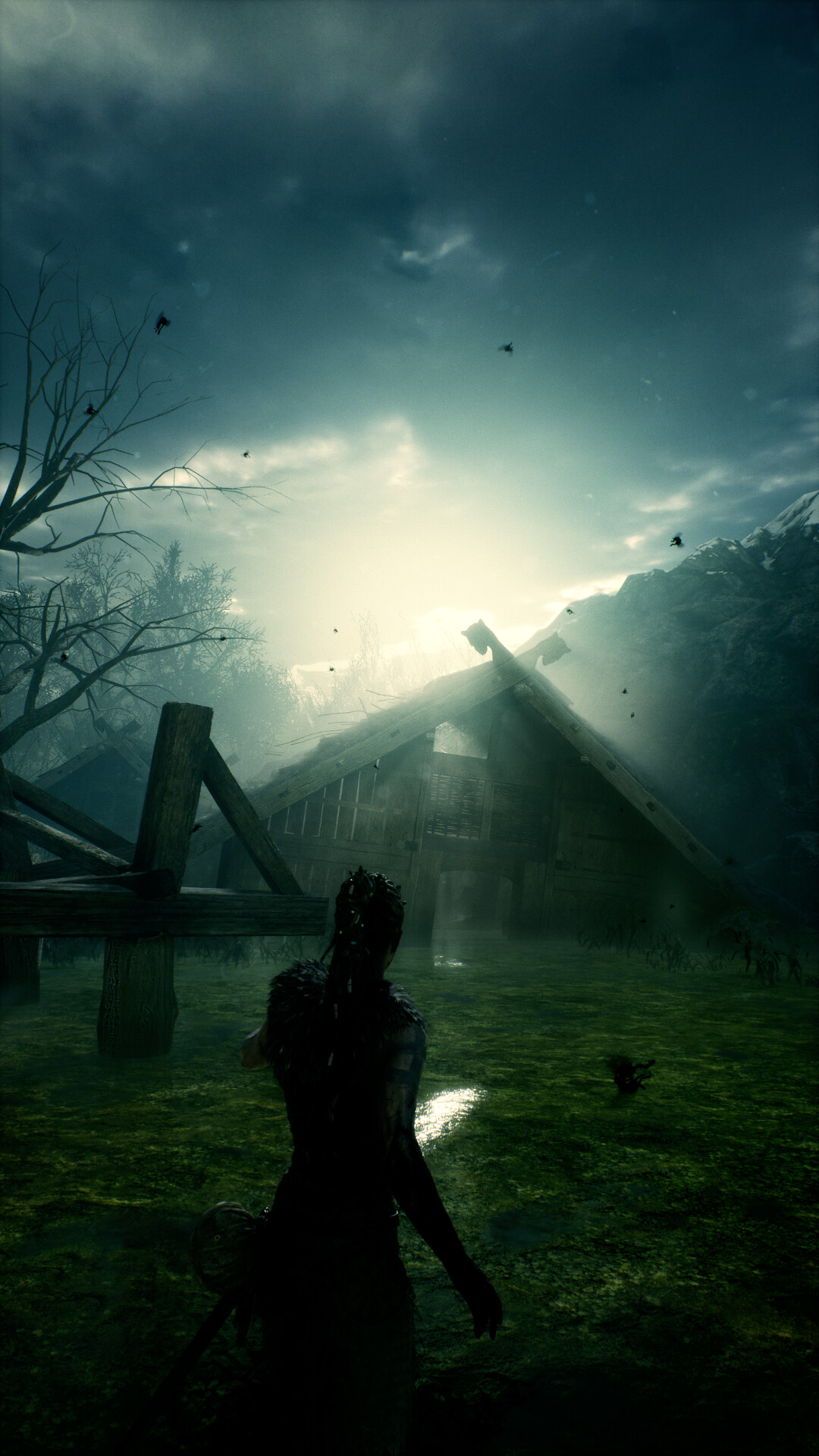This image appears to be a screenshot from a video game, showcasing a scene with computer-animated graphics. The entire image is saturated with a grayish-blue hue, enhancing its atmospheric mood. In the background, a cloudy sky lets through a bit of sunlight, casting a soft glow over the scene. The light highlights a wooded area and a partially caved-in, brown wooden A-frame house with a section of a wooden fence to the left. To the right of the house, there's a skeletal wooden structure, consisting of bare poles and a flat floor. The scene features a large lawn with green grass and trees in the background. Dominating the bottom center of the image is a dark silhouette of a woman, her back turned. While her features are unclear due to the blurriness, she appears to have beads in her braided hair, which is pulled back. She is dressed in a black fur vest, and a sword is visible on her left side. The detailed composition and lighting create a captivating and immersive outdoor setting.